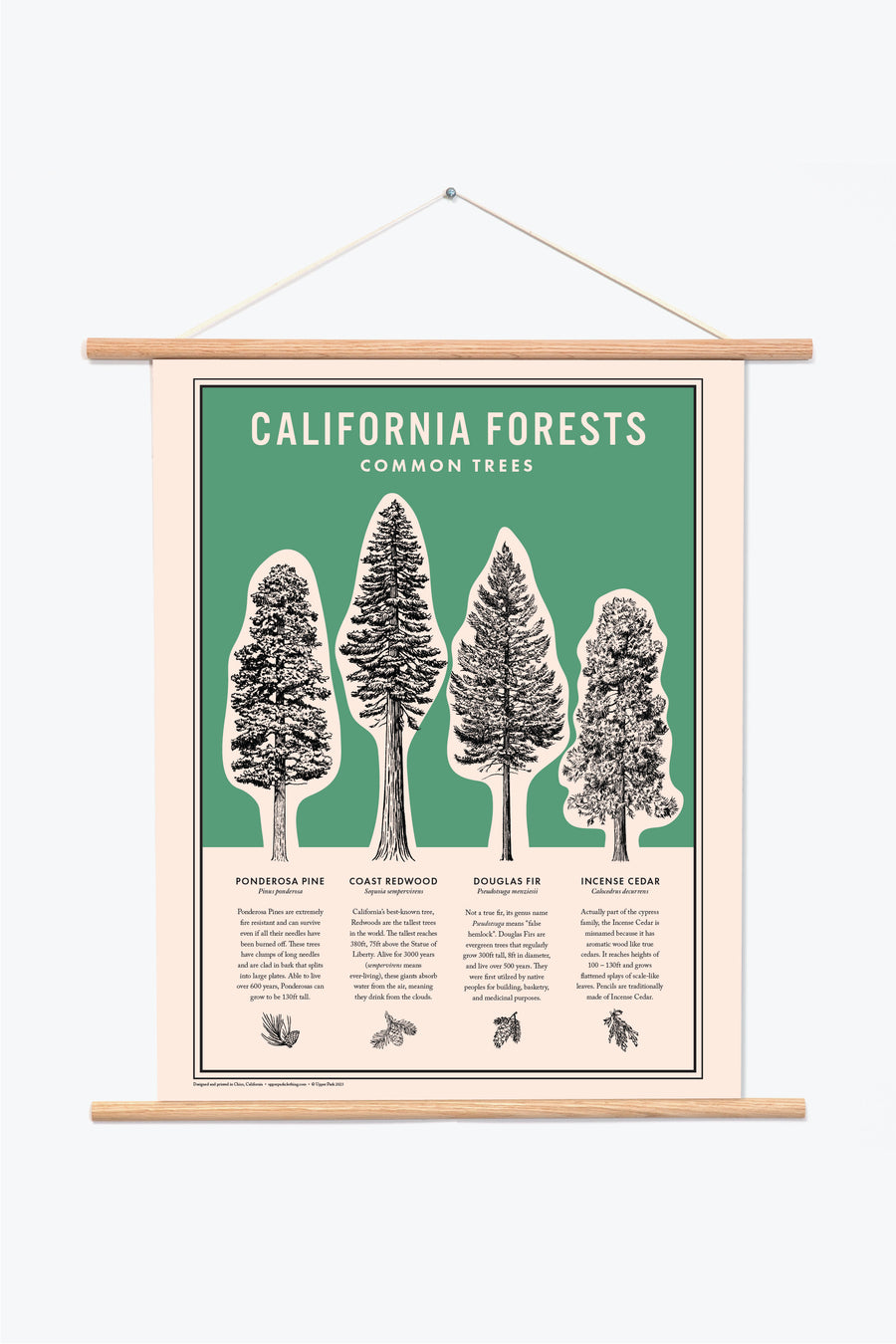The image depicts a hanging scroll with a beige-colored background, suspended by a beige string from a silver nail on a white wall. The scroll is framed at the top and bottom by light wooden rods, and the main segment of the scroll is colored in forest green with a beige border. At the top of the scroll, it reads "California Forest, Common Trees" in a beige-colored font.

Below the title, the scroll features black-and-white depictions of various trees set against the green background. The trees depicted include the Ponderosa Pine, Coast Redwood, Douglas Fir, and Incense Cedar. Each tree is accompanied by text that describes its unique characteristics. For instance, the Ponderosa Pine is noted for its extreme fire resistance and ability to survive even if all its needles have been burned off. The text mentions that Ponderosa Pines have clumps of long needles and bark that splits into large plates.

The bottom section of the scroll provides additional information about each tree, including illustrations of their respective pine cones. Despite some difficulties in reading the blurred text, the scroll offers a visually informative display about common trees found in Californian forests.